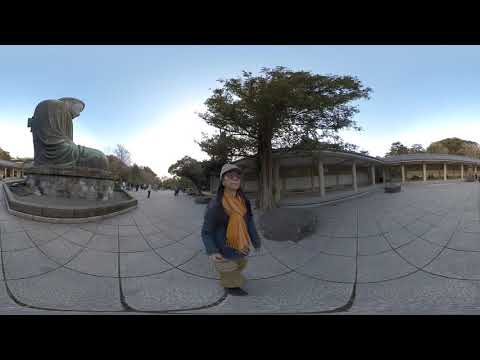This panoramic image captures an expansive, historical courtyard with a serene, monumental Buddha statue centrally positioned on a platform. The area is defined by its concrete tiled ground, which features geometric marks. Dominating the foreground is a solitary figure, an older Asian woman, sporting a dark blue jacket, a thick orange scarf, khaki pants, a gray cap, and glasses. Due to the panoramic nature of the shot, some distortion makes her appear slightly squashed.

Behind her, a tree stands prominently near a rounded building adorned with white pillars, extending to form an L shape around the courtyard. The building appears to have an awning supported by columns, offering a sheltered walkway. The scene, set under a clear sky, also features other distant figures scattered throughout the plaza, adding life to this historical site.